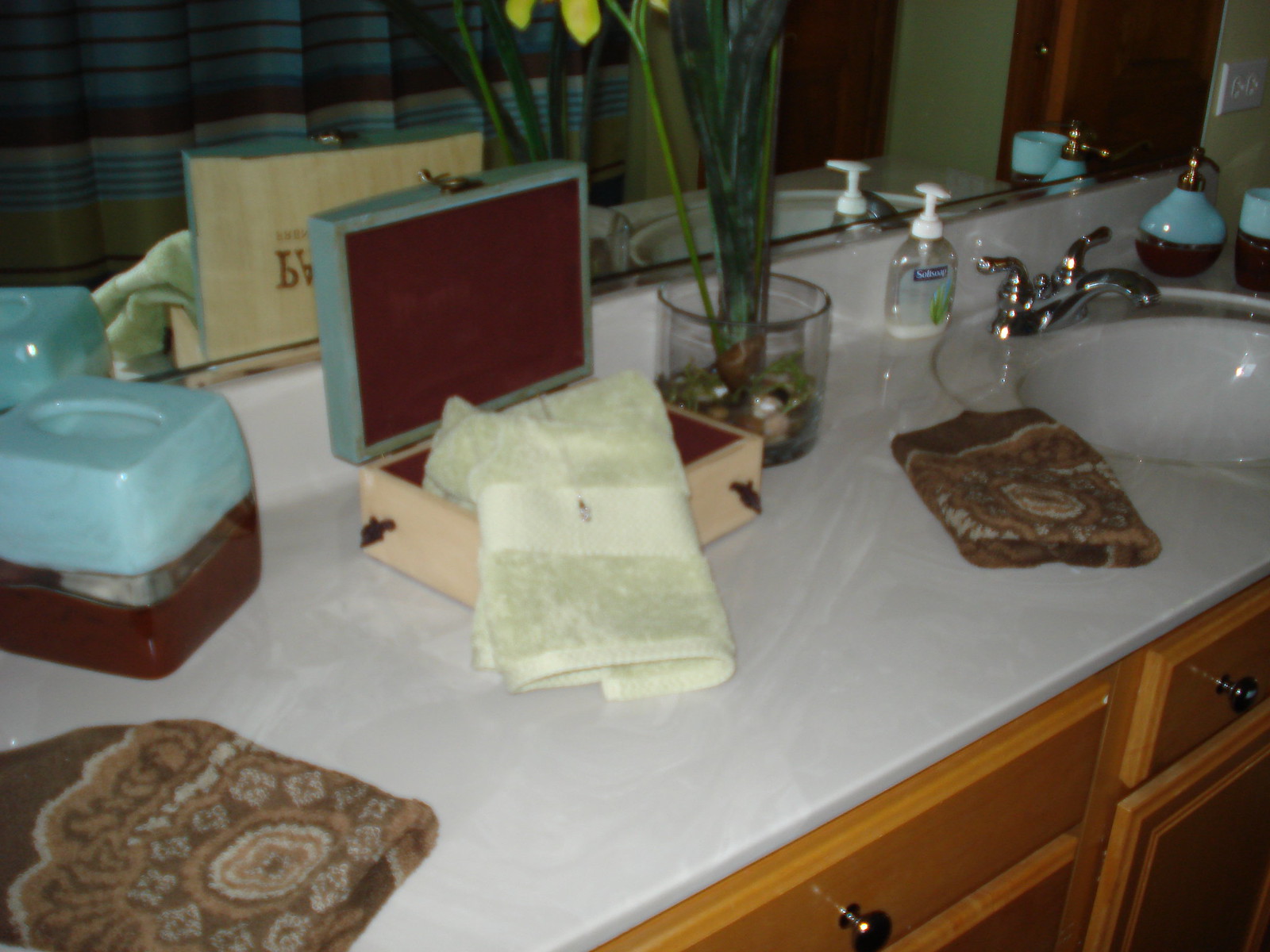This image showcases a meticulously organized and immaculately clean bathroom. The centerpiece is a long, solid white countertop integrated with a sink. Below the countertop are light brown wooden cabinets, each adorned with two silver knobs. 

On the countertop, to the left, are two neatly folded brown towels with a delicate light-colored floral design. Central to the arrangement is a small, open jewelry box with a white towel draped over its edge. The box boasts a luxurious dark maroon, likely velvety interior, with a beige bottom and a light blue lid.

Adjacent to the box on the left is a tissue holder, composed of a brown base, a translucent middle section, and a blue plastic top. On the right side of the box stands a clear cup displaying tall green stems topped with vibrant yellow flowers. Further to the right, closer to the sink, is a bottle of basic liquid hand soap.

To the far right of the sink, two items sit side by side: a cup and a soap holder. Both items feature a consistent design theme with a brown base, a clear middle section, and a blue top, matching the tissue holder.

The pristine backdrop includes a large, spotless mirror reflecting a shower area. The visible shower curtain is adorned with a sophisticated pattern comprising blue, white, and brown stripes. Completing the scene is a dark wood door, blending seamlessly with the other wooden elements in the bathroom.